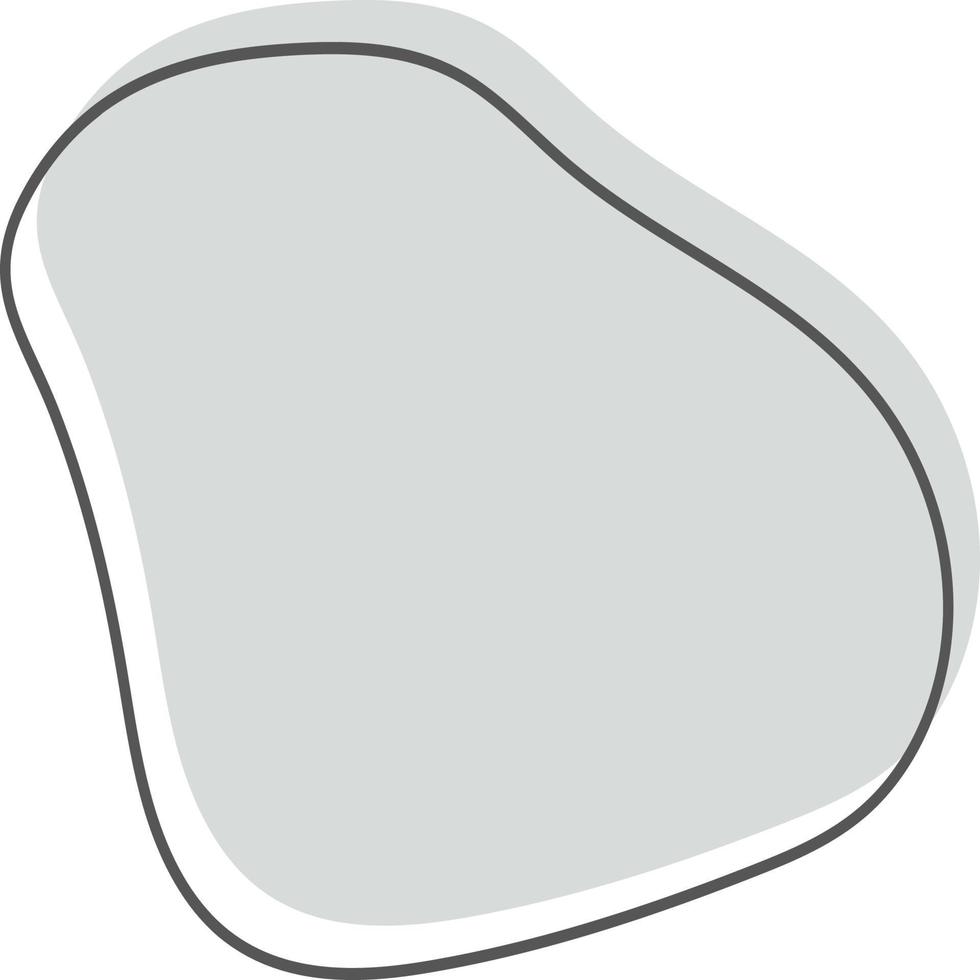The image on the screen depicts a digitally created, highly clean outline of an oblong shape reminiscent of a lima bean with a distinctive square corner on one end. This shape is outlined in a bold, dark gray line, forming an hourglass-like curve, with the top end narrower than the bottom. Within this dark outline, another shape mimics the outer contour, filled with a light gray color. However, this inner shape is slightly offset towards the upper right, creating a white band that traces from the thick, dark outline on the top corner, around the curve, and down to the right corner. The overall effect is a sharp contrast between the flat light gray fill, the prominent dark gray outline, and the pristine white background.